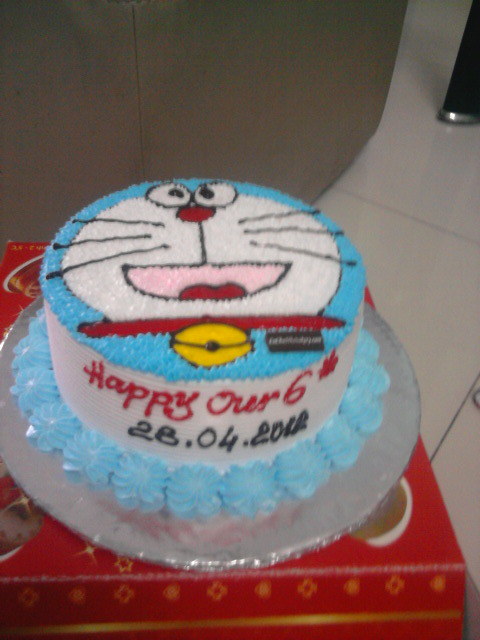This detailed photograph showcases a colorful birthday cake designed to look like the beloved cat character Doraemon. The cake is predominantly blue, white, red, and yellow. The character's face is skillfully crafted on the top, featuring a white inner circle with two large googly eyes, a red nose, a smiling mouth, and three whiskers on each cheek. A red collar with a golden bell adorns the bottom of the face. The text "Happy Hour 6" is written in red on the side of the cake, likely indicating the celebration of a six-year-old's birthday, and beneath it, the date "28.04.2012" or "26.04.2012" is inscribed in black, though the writing is slightly hard to discern. The sides of the cake are white with fine horizontal lines, and a ring of blue icing circles decorates the base. The cake sits on a silver foil tray which is placed on a red and gold platform, captured at a top-down angle, and slightly leaning to the left.